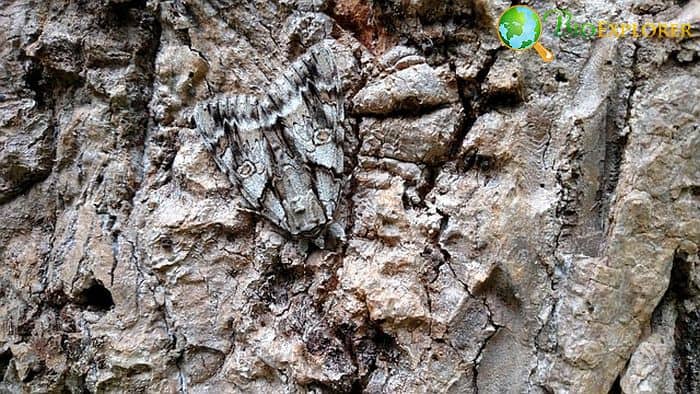This image, taken outdoors, captures a close-up of a rugged surface that appears to be part of a cliff or mountain rock formation, perhaps resembling a cave-like structure. The rock is primarily a blend of gray, beige, and tan hues, featuring jagged textures and cracks. Intriguingly, the surface contains markings that eerily resemble a face or mask with two eye-like shapes and a small mouth. The "mouth" area appears dented, creating an irregular head shape that makes it difficult to determine whether the face is intended to be human or animal. The face-like pattern, possibly carved or naturally occurring, blends into the rock but also mildly stands out due to the color variations. Additionally, there's a hint of yellow and green in the upper right part of the image, possibly containing text and depicting a globe, suggesting human interaction or signage around the area. This scene evokes the mystery of natural formations and the tendency of our eyes to find familiar shapes in the environment.